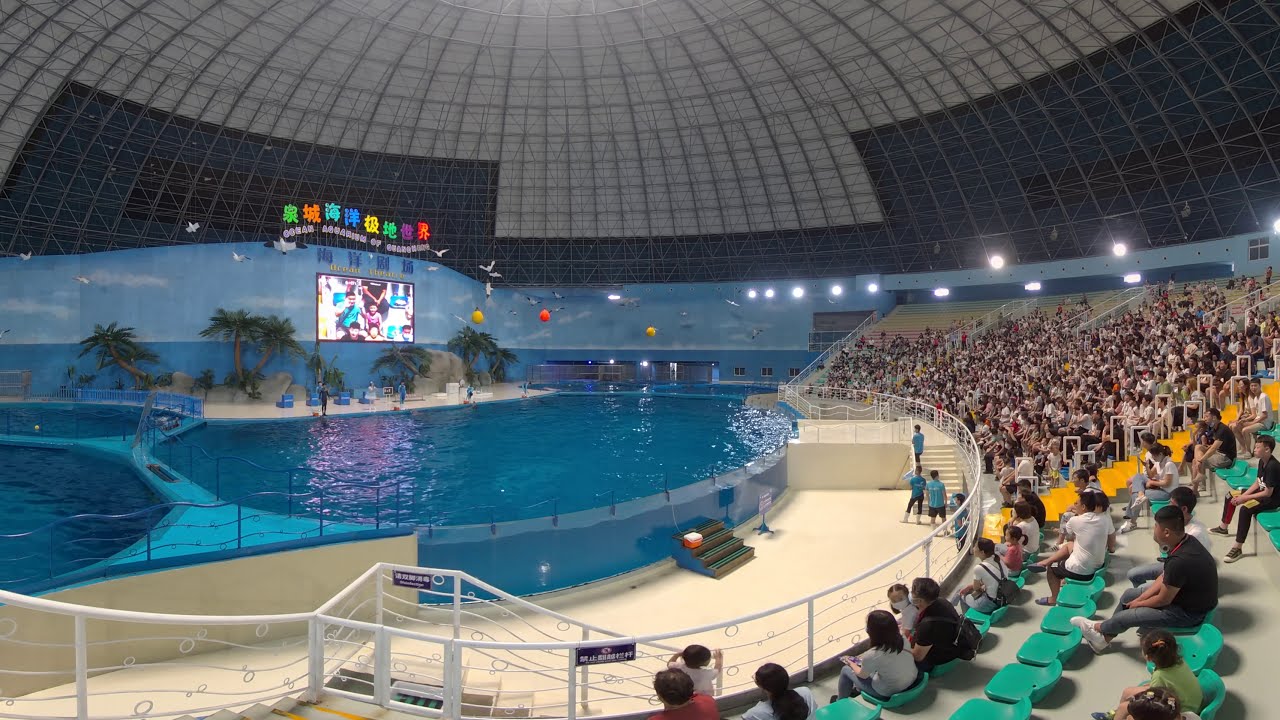The photograph captures an indoor aquatic stadium, reminiscent of SeaWorld, likely located in an Asian country given the large video board displaying rainbow-colored text in an Asian script, possibly Chinese or Japanese. The stadium is enclosed within a blue and light gray dome. Turquoise-colored pools of clear blue water are situated on the left, with a white walkway and steps leading up to the pool, presumably for trainers and staff. On the right, rows of yellow seats filled with a diverse crowd in casual attire—black, white, pink shirts—extend upwards in stadium-style seating. An orange Gatorade cooler is positioned at the bottom left. Above a small stage behind the main tank, a giant monitor zooms in on two crowd members, framing the scene as spectators eagerly await a performance, perhaps involving Killer Whales, seals, or dolphins.